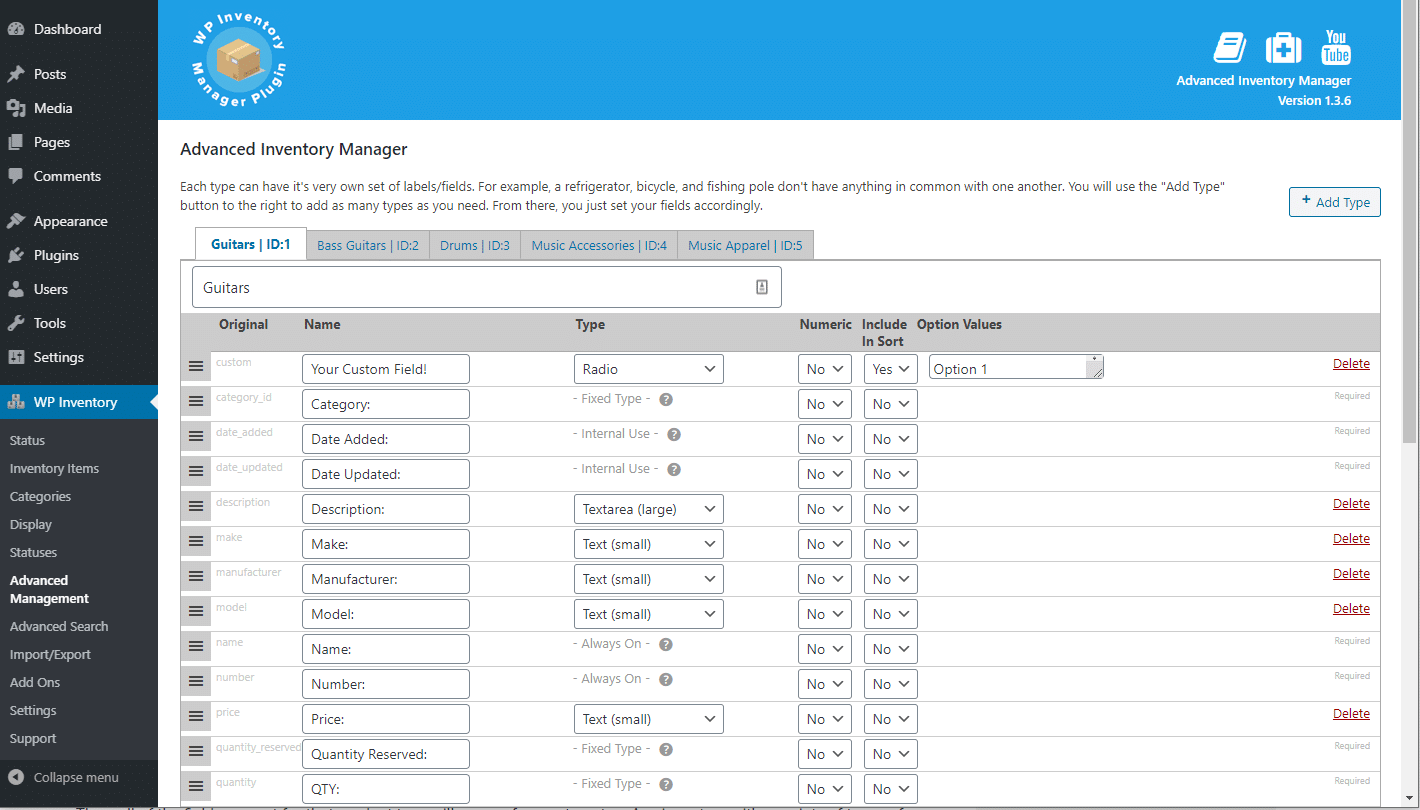This screenshot showcases the interface of the WP Inventory Manager plugin. The page is bordered by a prominent black line vertically down the left-hand side and a blue bar horizontally across the top. The main content area below the blue border features a white background with black text for a clean and straightforward display.

In the upper right-hand corner of the page, the text "Advanced Inventory Manager version 1.3.6" is prominently displayed. Adjacent to this text are three icons: a book icon, a medical icon, and a YouTube icon, providing quick access to relevant resources and information.

On the left sidebar, which is shaded in light gray, there is an extensive menu comprising various options. The menu items are listed in the following order: Dashboard, Posts, Media, Pages, Comments, Appearance, Plugins, Users, Tools, Settings, WP Inventory, Status, Inventory Items, Categories, Display, Statuses, Advanced Management, Advanced Search, Import, Export, Add-ons, Settings, Support, and Collapse Menu.

Overall, the WP Inventory Manager plugin interface is well-organized, offering users a comprehensive range of options and tools to manage their inventory efficiently.